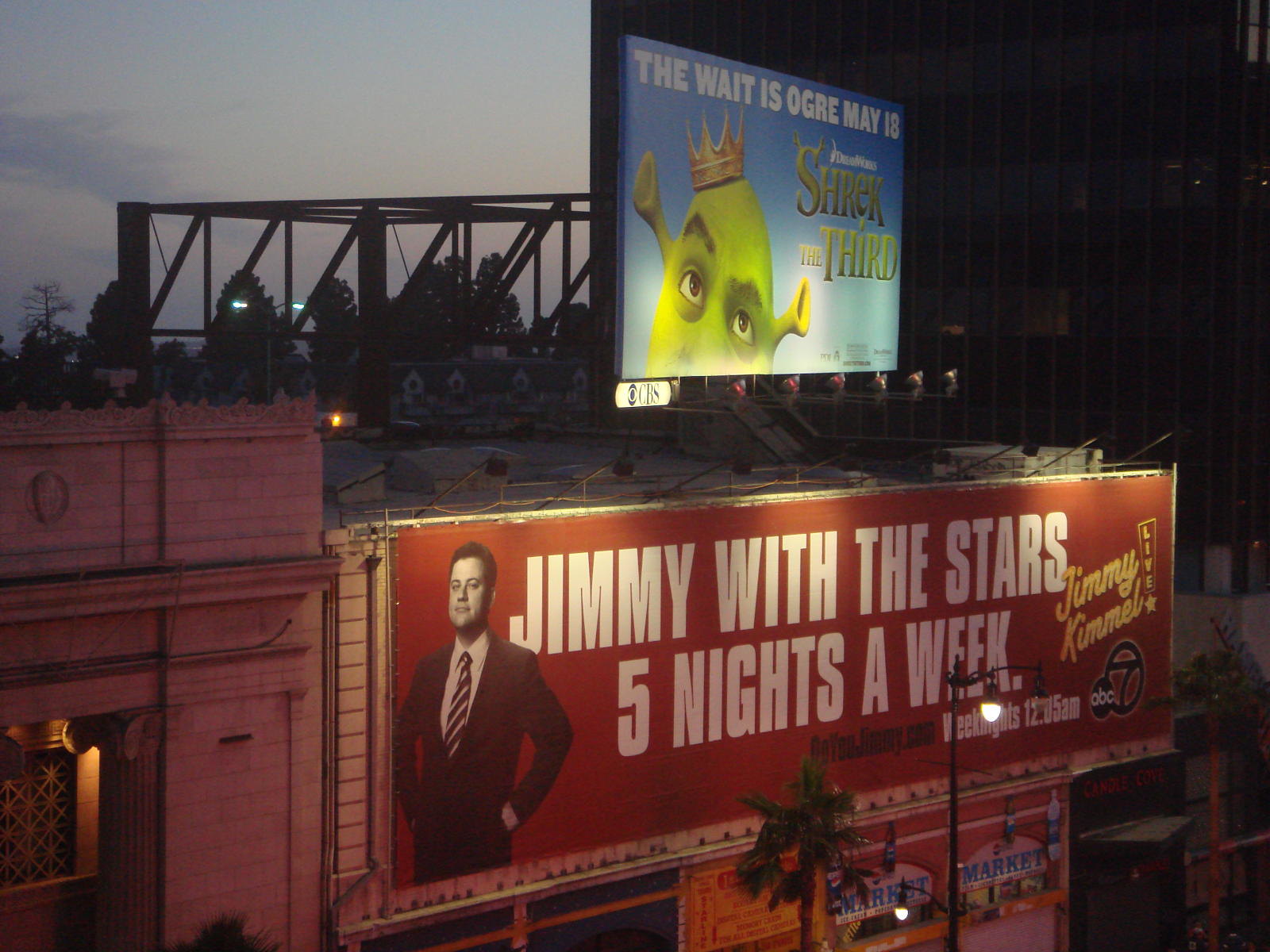In this outdoor photograph, the sky in the upper left corner suggests it is either dusk or dawn, casting a soft light over the scene. The background features trees and a cityscape below, with the tops of buildings lining the horizon. Prominently, atop one building, a rectangular sign reads "Jimmy with the stars five nights a week." Above this, a large billboard announces "The wait is over May 18th Shrek the Third." In the foreground, streetlights illuminate the area, where a palm tree and the edge of another building are also visible, adding to the urban environment.